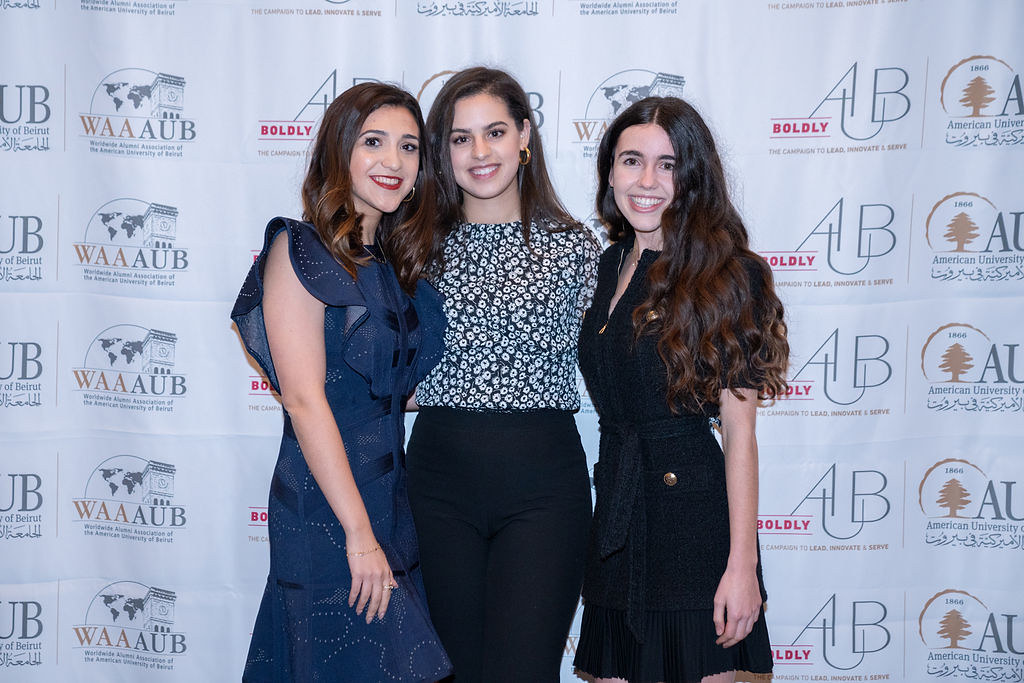This photograph shows three women posing closely together and smiling at the camera, standing centrally from about the knees up. The woman on the left is wearing a long blue dress with lacy patterns and a flared shoulder design, complemented by dark red lipstick and brown hair that falls just below her shoulders. The middle woman, dressed in a black high-waisted pants paired with a blue and white floral-patterned shirt, has light skin and wears gold hoop earrings. The woman on the right sports a short, dark blue or black dress with gold buttons and a ribbon, her very long, curly brown hair cascading almost to her waist. All three women have light skin. Behind them is a white billboard plastered with various company logos, including one prominently featuring the letters "A" and "B" alongside the word "boldly." Another logo includes a globe with the text "W-A-A-A-U-B" and mentions "The American University." The image captures the women in a joyful moment, with their attire and the detailed backdrop suggesting a formal or celebratory event.